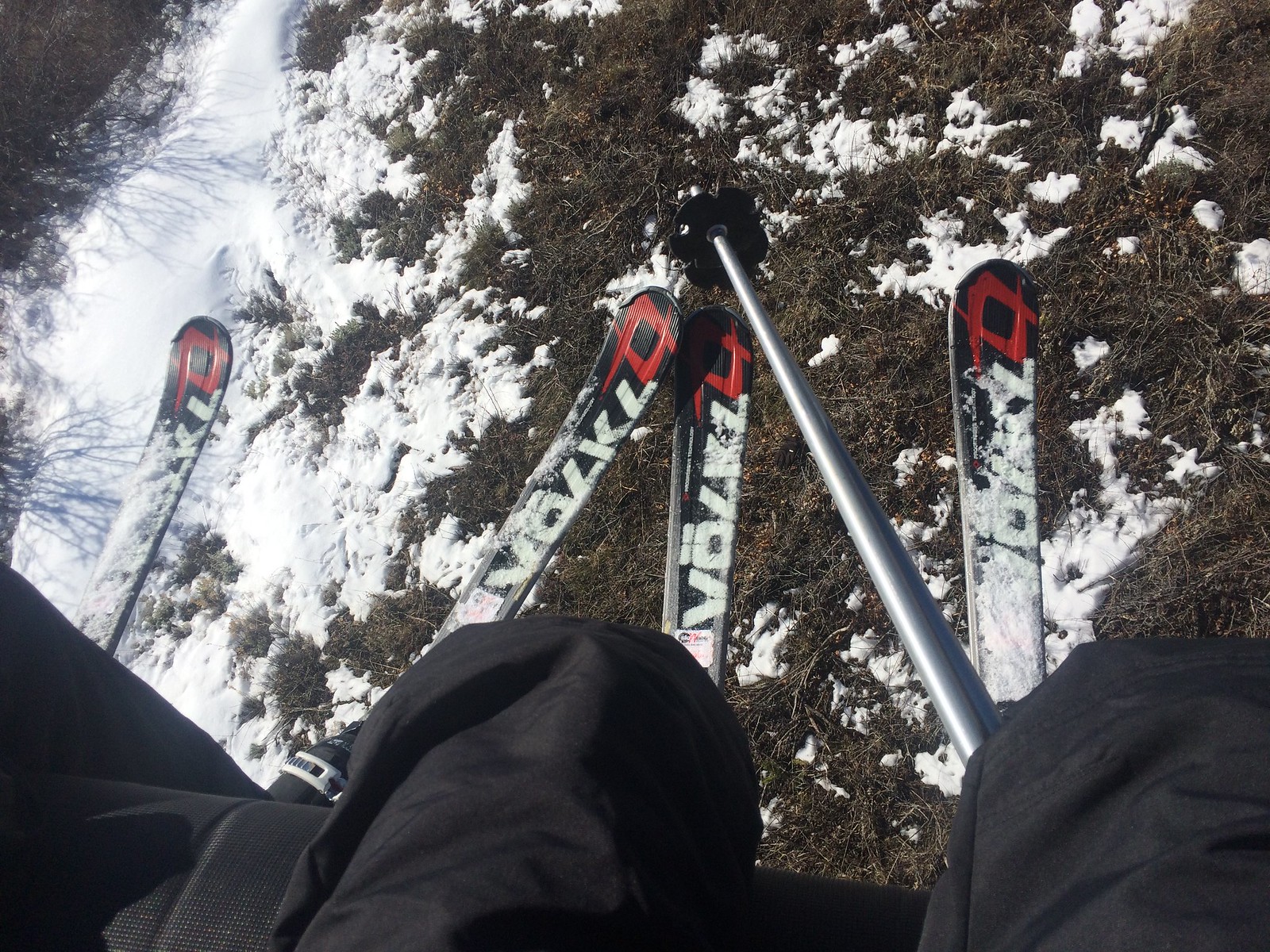This vibrant color photograph captures an aerial view from a skier's vantage point on a ski lift ascending a mountain. The foreground prominently features the skier's knees, clad in black pants, nested against a black seat running along the bottom. Spread underneath them are four black skis, each branded "Volk" in white letters with a distinctive red logo at the tips. The scene below presents a mix of grassy terrain dotted with patches of snow, transitioning to more densely snow-covered areas on the left, where shadows of pine trees, their branches dusted in snow, cast intricate patterns. The image conveys a serene yet dynamic moment as the lift transports skiers towards higher elevations with more substantial snowfall, ideal for skiing.